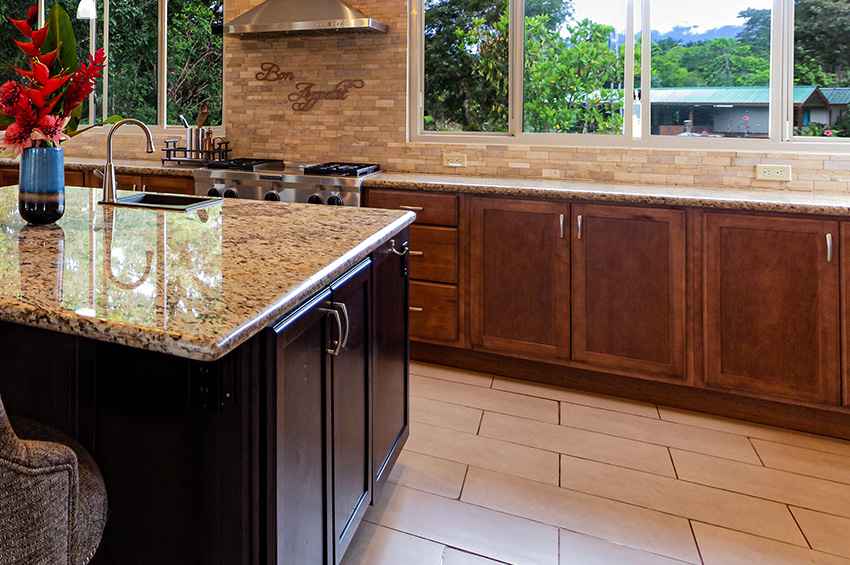This image captures a well-lit kitchen with a light tan tile floor, featuring rectangular-shaped tiles that resemble floorboards. The centerpiece is an island counter located towards the left center of the image, equipped with a sink and a granite countertop that showcases a speckled pattern of brown, black, and beige. The island's base is a dark brown color and includes a padded, dark gray bar stool. To the right of the island, there are dark brown or black cabinets extending towards the back wall, accompanied by lighter brown cabinetry beneath a set of large sliding windows. Through the windows, a tree-filled, green landscape and distant houses are visible, indicating daylight. On the marble countertop near the sink sits a blue flower pot with red flowers. The back wall features a vent hood above a cooking range, and a charming sign reading "Bon Appetit" is mounted on a wall adorned with a brick design. Various kitchen utensils, cabinets, and drawers in varying shades of brown complete the setting, contributing to the kitchen's warm and inviting atmosphere.